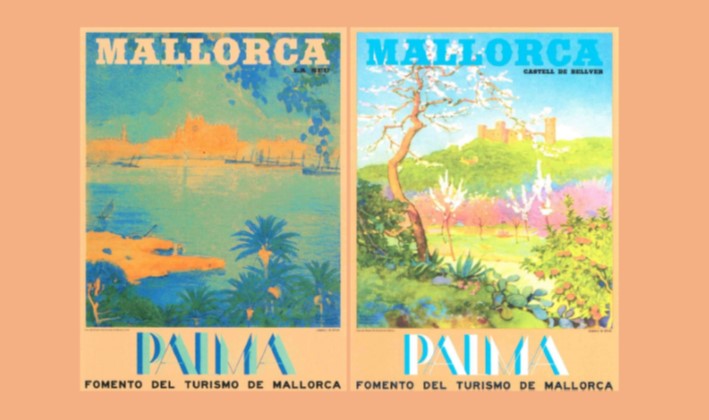This horizontal image showcases two adjacent, vintage travel posters for Mallorca, their edges slightly worn and the paper yellowed over time. Both illustrations rest on a light orange background, echoing a nostalgic charm. Each poster is crowned with the word “Mallorca,” and, at the bottom, the words “Palma, Fomento del Turismo de Mallorca” assert the promotional purpose.

The left poster features a serene coastal scene, with rugged hills or cliffs overlooking a tranquil bay. Blue palm trees accent the lower right corner, while the top showcases the word “Mallorca” in bold white letters. 

Contrasting the coastal vibe, the right poster presents a lush landscape dominated by green hills and foliage. A historic castle rises in the background under a clear blue sky, accompanied by vibrant pink and white flowers melding with the verdant greenery. The word “Mallorca” appears in blue letters, paralleling the left poster's layout.

The posters collectively embody the charm and allure of Mallorca, merging scenic vistas with historic landmarks, captured in muted pastel hues that evoke a sense of timeless travel nostalgia.